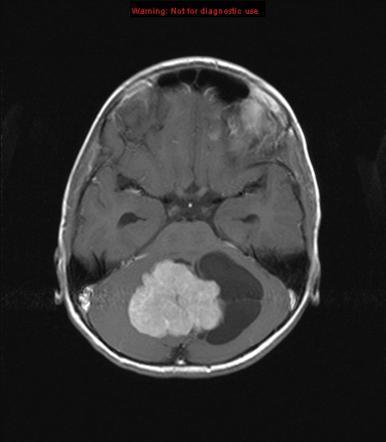The image depicts a black and white scan of the interior of a skull, presented against a completely black rectangular background. In the center of the image, there is an oval or egg-shaped section, outlined in white, showing detailed grayscale sections of a brain. The brain is visibly segmented into various lobes, with dark, light gray, and black regions that reflect the organic, fleshy texture of brain matter. Notably, there is a large white mass in the center, which could be indicative of a tumor or other abnormality. At the top of the image, there is a small piece of red text that reads "warning, not for diagnostic use."